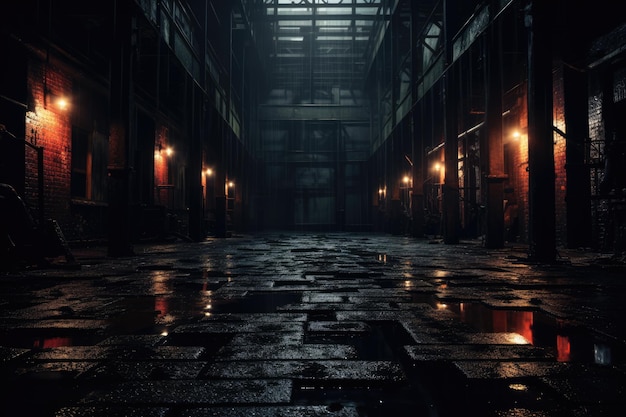This evocative nighttime photograph, taken from a worm's eye perspective close to the ground, portrays a long, possibly warehouse-like room or covered alley. The symmetrical, low-angle view faces directly down the center, where a damp, black brick or stone floor extends, reflecting the aftermath of a recent rain. The scene is predominantly dark, with minimal skylight filtering through the windows and faintly illuminating parts of the blackened ground. Orange-yellow lights are set up in regular intervals along the brick walls, casting glows that reflect off puddles and damp surfaces, enhancing the industrial and grungy atmosphere. The photograph showcases a second level, supported by pillars, adding to the mystery and depth. On both sides, the walls appear to house regularly spaced lights, reminiscent of doorways or porch lights, suggesting an abandoned urban setting. The street-like floor may lead to a dead end, featuring an upward incline or a continuation to an underpass. No people or text are visible, emphasizing the eerie solitude and timelessness of the scene.